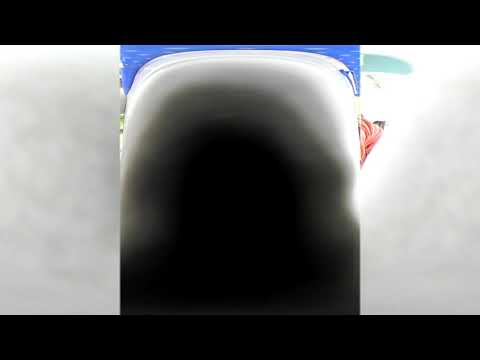The image is an extremely distorted attempt at a panoramic shot with various elements that appear ambiguous and disjointed. Dominating the center is a white rectangular shape transitioning from black to gray and white, capped with a sea-blue hue at the top. This central area also features an abstract white blob with a dark black core. On the right side, there are notable grayish-white blobs, one of which contains a pink or reddish feature resembling electrical cables or an extension cord.

Further right, a small section appears to depict the nose of an animated bear, reminiscent of characters in a 1950s children's storybook, marked by its black nose and brown fur. Flanking the entire scene are white bars on either side, with the right one also encompassing part of the bear's feature. The blurry and somewhat indistinct layout is bordered on the top and bottom by black bars, adding to the unclear and fragmented nature of the picture. An animated-looking blue area, suggestive of the sky, tops the entire image. The visual disarray suggests it might be a close-up screen grab of a larger video taken out of context.